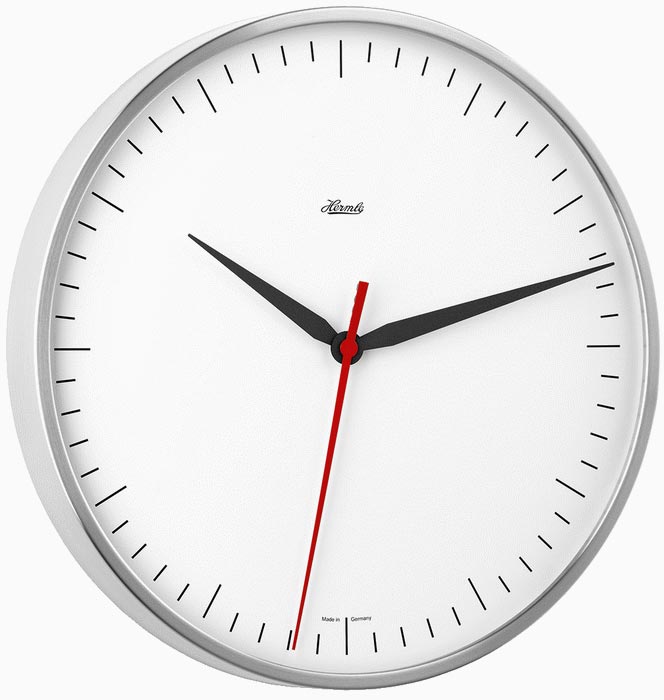A detailed image of a round clock is depicted, possibly originating from a computer-generated design rather than a photograph. The clock features a white outer casing with a subtle silver lining on the inner edge. Instead of traditional numerals, the clock face is adorned with minimalist dashes representing the hours. The clock hands include a black hour and minute hand, contrasted by a striking red second hand. A cursive brand logo is present near the top of the clock face, though it is not legible. At the bottom, in very small print, the clock is marked with the words "Made in Germany."